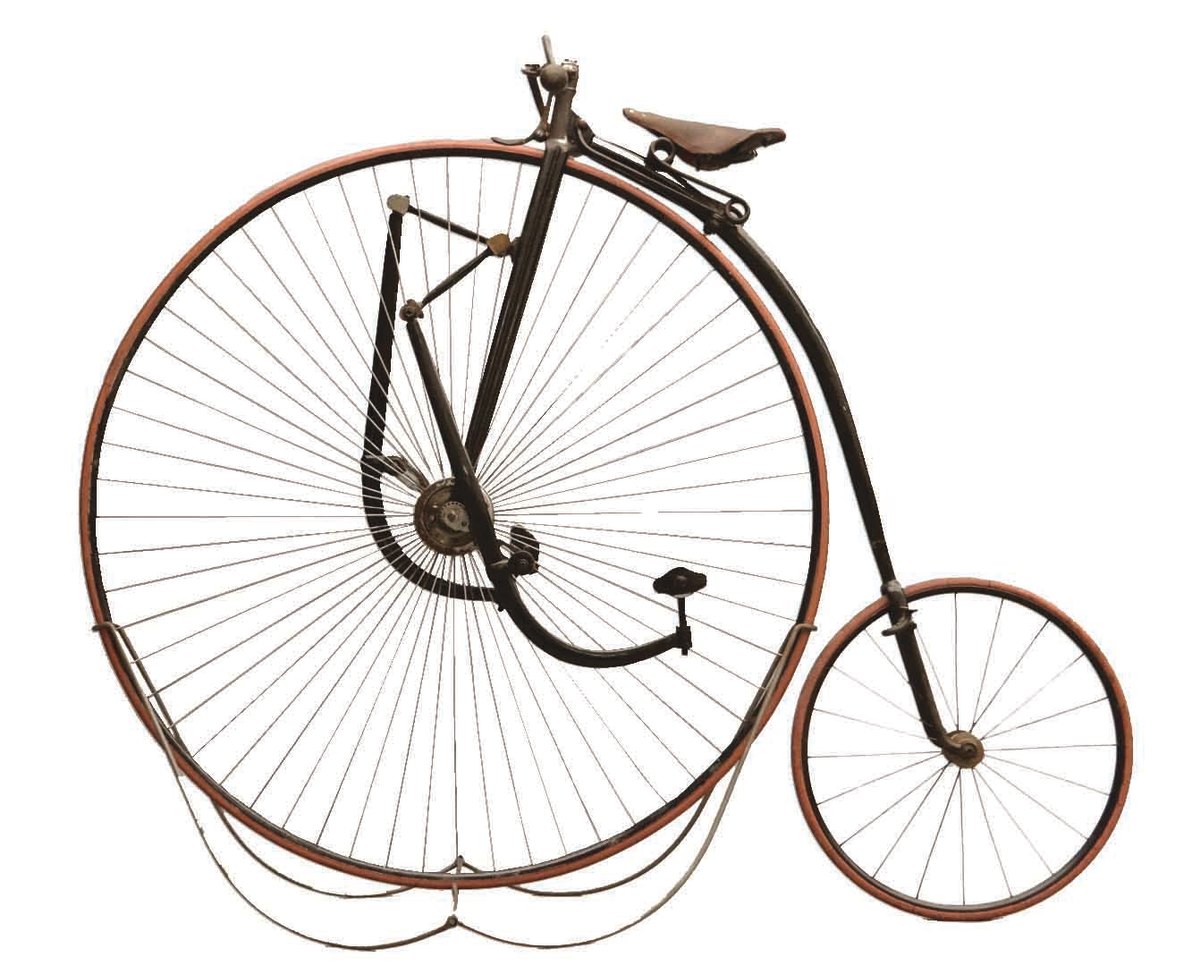This is a detailed photographic image of an antique Penny Farthing bicycle, a design popular in the late 1800s. The bicycle features a very large front wheel and a much smaller rear wheel, reflecting its distinctive style. The front wheel, which dominates the structure, has numerous dark brown spokes and is mounted on a stand for support. The foot pedals are directly attached to the hub of this large front wheel, integrated into a gear assembly connected to the steel fork that extends upward to the narrow handlebars. The handlebars are brass-like and positioned close together.

The seat, situated high above the large front wheel, is narrow and made from brown leather, supported by a spring mechanism for added comfort. The bicycle's frame has a dark brown or black hue, with the aging metal showcasing carbon deposits that give it a weathered, historical appearance. The smaller rear wheel has fewer spokes and is connected through a long metal bar extending from the frame.

The entire bicycle stands out prominently against a clean, white background, emphasizing its antique characteristics and making it clear that this is a preserved piece, likely displayed in a museum. The overall appearance and unique design underscore its historical significance and the engineering challenges of its time, portraying the Penny Farthing as both a remarkable innovation and a difficult, potentially dangerous mode of transport from an era long past.